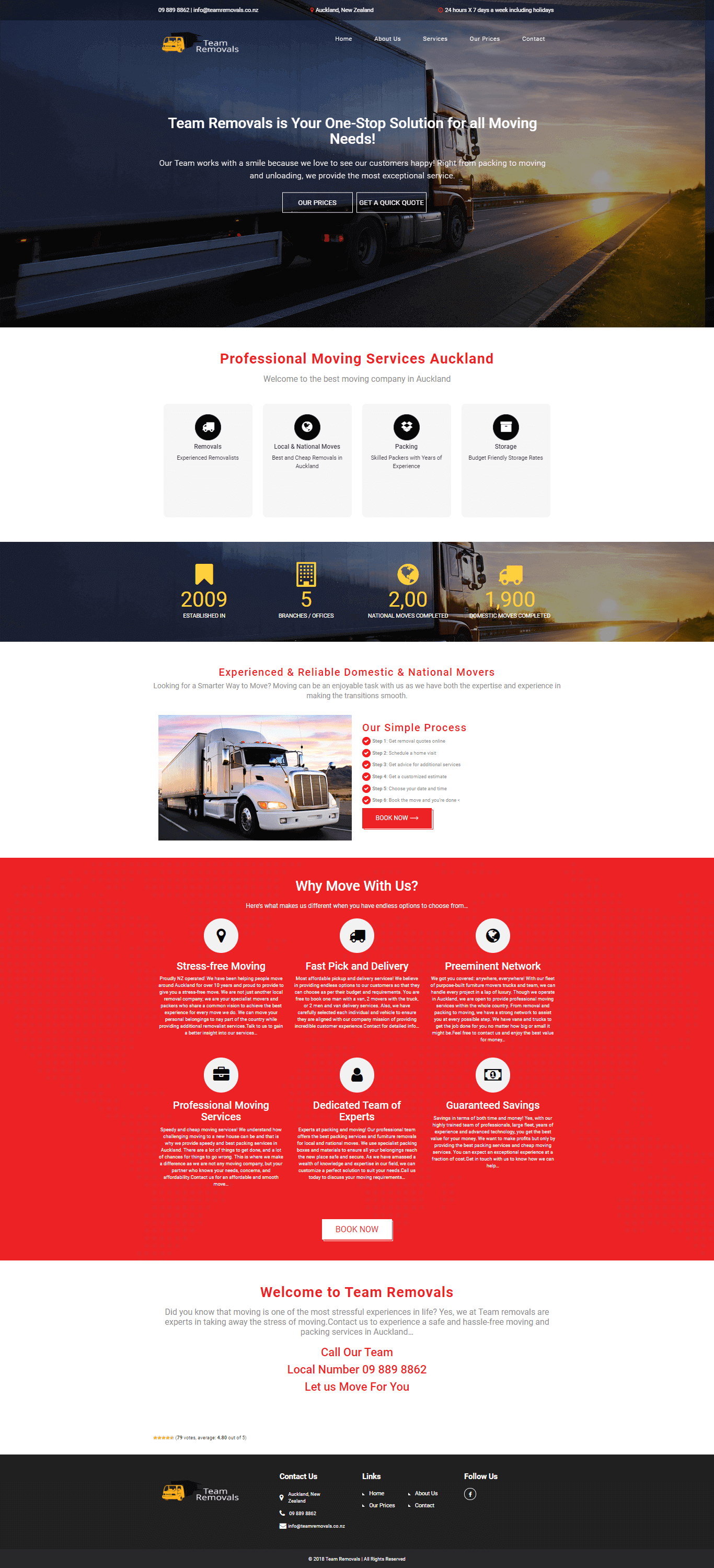The image is a vertical, triangular-shaped screenshot, likely taken from a website due to its elongated format, making the text within it difficult to read. At the top of the image is a horizontally oriented photo of a semi-trailer truck driving down a road into the sunset. Superimposed on this image is text reading, "Team Removals is your one-stop solution for all moving needs." There is other unreadable text overlaying the photo.

Below this section, on a white background, the text "Professional Moving Services" is clearly visible, followed by "Auckland." There are also four side-by-side icons that are selectable but not clearly identifiable due to their small size.

Further down, there is a narrower, horizontally rectangular cropped image of the same semi-trailer truck driving into the sunset. This section features icons accompanied by numbers: "2009," "5," "2.00," and "1900." Unfortunately, the accompanying explanatory text is too small to discern, leaving the significance of these numbers ambiguous.